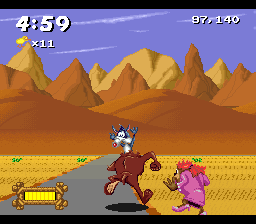A vibrant, small square screenshot captures a lively moment from a video game featuring beloved Looney Tunes characters in a desert setting. Dominating the scene, a gray pathway winds through the sandy terrain that stretches across the image's left and right peripheries. Center stage, the Tasmanian Devil—seen from behind—is in hot pursuit of the frantic Wile E. Coyote, who faces forward with arms raised in alarm. Trailing closely behind, a pink character's back is visible in the lower right portion of the scene. A yellow progress bar is situated in the bottom left corner of the image. At the top of the screen, time played is displayed, with a multiplier of "x11" just below. Meanwhile, in the top right corner, the player's score is prominently featured.